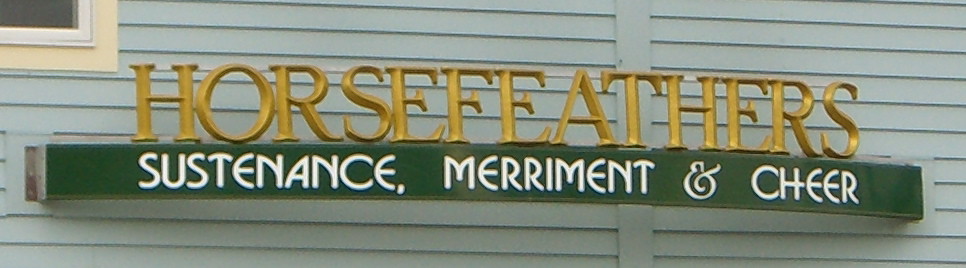The image showcases a building with green siding or wood paneling. Prominently displayed over the entrance is a sign with bold, gold, all-capital letters spelling "HORSE FEATHERS." Directly beneath this sign is a long, rectangular one featuring a deep green background with the words "sustenance, merriment, and cheer" in elegant white text. In the upper left corner of the building, there's a window framed first by a beige border and then by a white inner frame, hinting at a dark interior. It's likely that this detailed signage is indicative of the building housing a restaurant or a place meant for dining and social gathering.